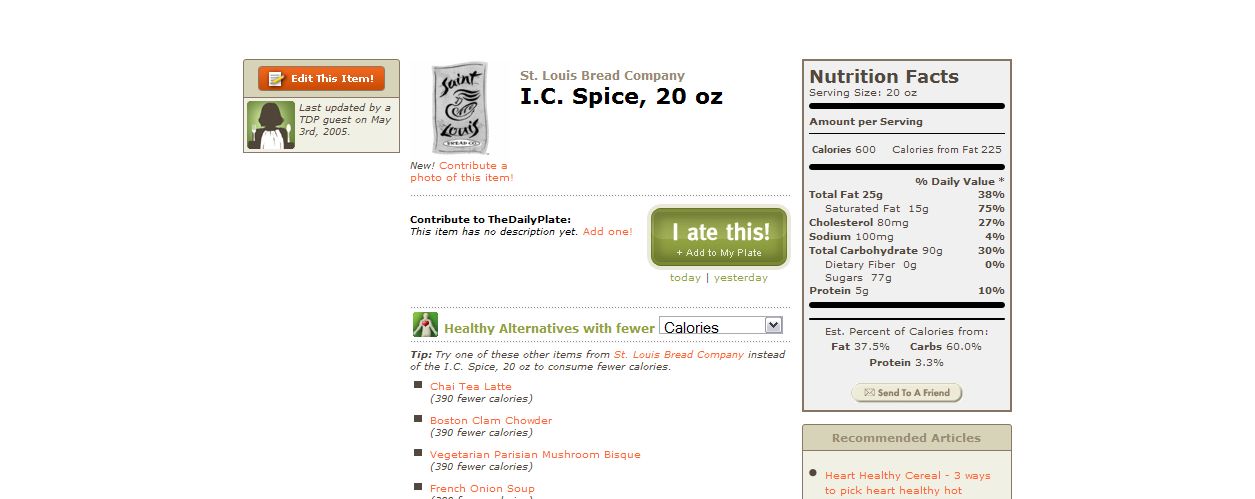This image appears to be a screenshot from a health or nutrition-focused app, potentially MyFitnessPal, showcasing the nutritional details of a product from St. Louis Bread Company, specifically "IC Spice 20 oz." The layout suggests it is a digital page on a website or app interface. At the center of the image, prominently displayed, is the product's name and description. 

To the left of this central block, there is an avatar of a woman along with some text, possibly indicating a review or user interaction section. Above this, it says “Edit this item,” with a note indicating it was last updated by a top guest on May 3rd, 2005, hinting that the image is quite old.

On the right-hand side, there is a detailed box listing the nutritional facts of the product, including various health metrics. This section also features links to recommended articles on heart-healthy cereals and tips for picking heart-healthy hot foods. 

In the middle, there's an interactive button, green in color, labeled "I ate this" which allows users to add the item to their daily consumption log. Below this, there is a prompt for contributing to a daily plate and a note stating the item has no description yet, inviting users to add one.

At the bottom of the image, a section titled "Healthy Alternatives with Fewer Calories" is visible, including a drop-down box for calories and various alternative food options listed below. Overall, the image is highly detailed, focusing on the nutritional content and user interactive features for documenting and managing dietary intake.